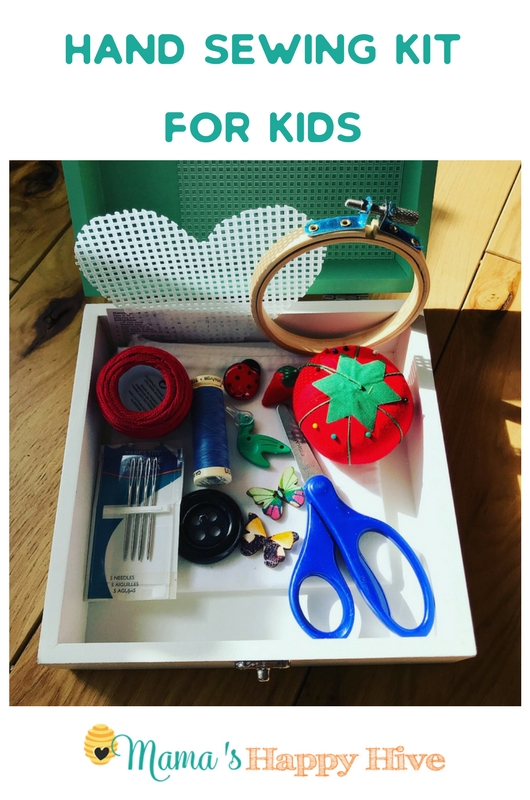The image captures an open, white sewing kit box with a green lid, placed on a brown floor. The top of the image features the text "Hand Sewing Kit" in green letters, with "For Kids" similarly inscribed below. Inside the box, on the left side, there are four sewing needles encased in a blue and white package. Adjacent to the needles, a circular red yarn ball is positioned. To the right of the yarn, there is blue sewing string laid horizontally, below which sits a large black button. Next to the button is a butterfly pin with black and yellow wings, and above it, a second butterfly pin with light green and purple wings. The top center of the box houses two ladybug pins, followed by a large red tomato pin cushion with a green top, located to the right. Below the cushion, there is a pair of scissors with blue handles. Various other small sewing trinkets, including a white heart with holes, are scattered inside the box. The bottom of the image displays the text "Mama's Happy Hive" with a small yellow beehive icon on the left, "Mama's" written in teal, and "Happy Hive" in orange.